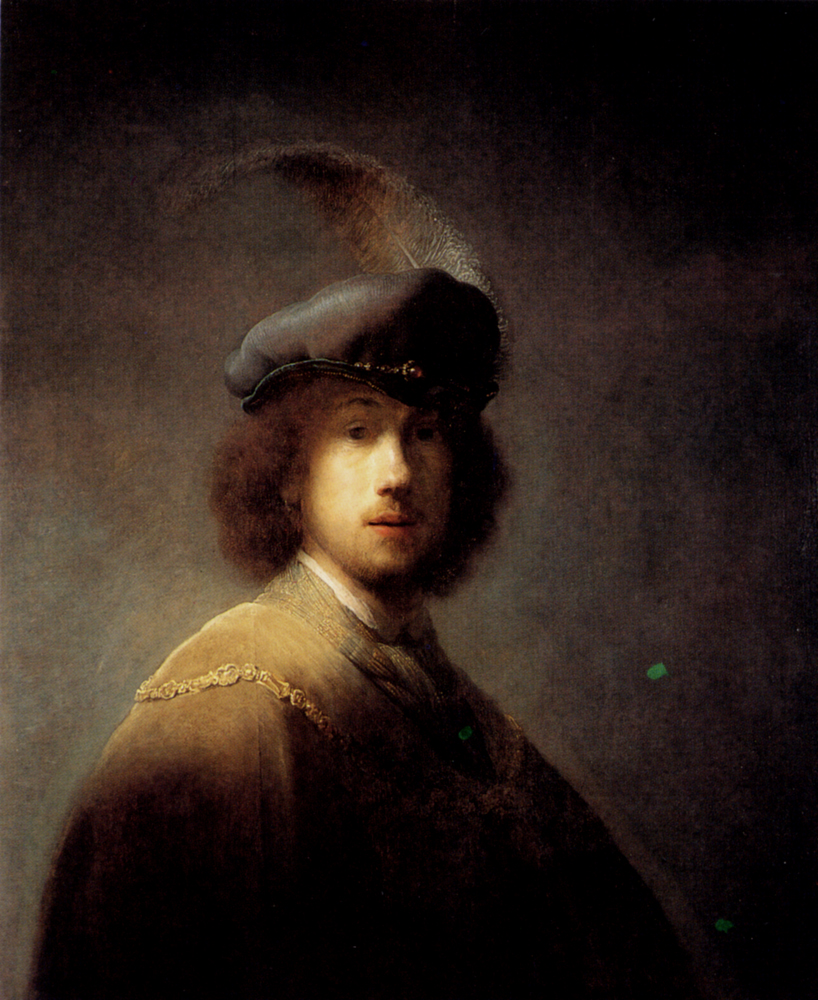This detailed oil portrait showcases a Caucasian man from a historical period, possibly the 1800s, characterized by his shoulder-length, curly, wavy brown hair. The man dons a distinctive, fluffy, black hat adorned with a large, brown, and grayish feather and a prominent red stone at the front. His pale face is oriented towards the viewer, though his body is turned to the right, creating a slightly surprised expression with his slightly open, full pink lips and small, close-set brown eyes. He sports a very light mustache with barely any beard. The portrait captures him in a rich, brown coat featuring gold designs across the shoulders, along with a slight hint of white from his undershirt at the neck. A subtle golden light illuminates his left side, adding depth to his attire. The background transitions from light brown near the subject to a dark, nearly black hue at the edges, enhancing the composition's overall dramatic and dark aesthetic. Two enigmatic green dots are visible towards the bottom right. The image is in portrait orientation, allowing for a detailed view from mid-chest level upwards.